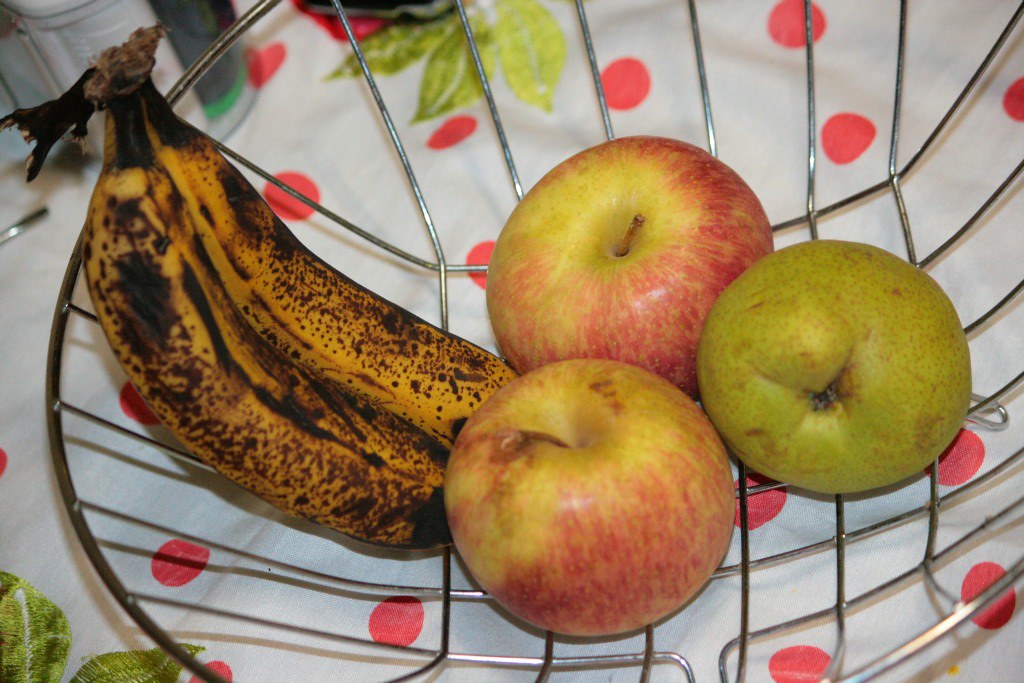In this photograph, a metal fruit bowl is prominently displayed at the center of a table, carefully arranged to prevent its contents from slipping through. The table is adorned with a red polka dot cloth that adds a touch of vibrant contrast to the scene. In the bottom left corner and partially towards the top left of the image, leafy elements are visible, contributing to a subtle, organic ambiance.

The fruit bowl contains two notably brown bananas, which are still connected at the stem; one banana has already been removed, leaving part of the stem exposed and extending backward. These bananas are at a stage of overripeness, ideal for use in banana bread.

Accompanying the bananas are three pieces of slightly aged fruit. On the top of the bowl lies a red apple tinged with green, complete with its stem. Below it, another apple, similarly colored and stemmed, shows signs of browning, especially noticeable near the top left. Nestled at the bottom is a green pear with brown spots, indicating it's well past its peak ripeness.

Additionally, a plastic container, partially visible in the background, holds items in shades of white, gray, and green. However, the fruit bowl with its aging contents captures most of the viewer's attention, symbolizing the passage of time and the ripening process of nature’s bounty.